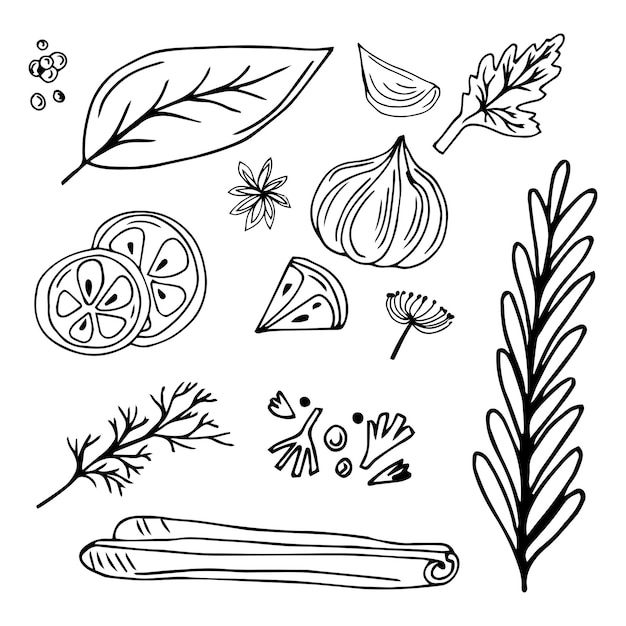This black and white illustration features an intricately detailed collection of various botanical elements, all rendered in pen or marker against a stark white background. The image prominently includes a range of vegetables, plants, and fruits, such as peas, a leaf, a citrus slice (either orange or lime), thyme sprigs, garlic, seeds, and pollen grains, resembling those you might find in a garden. Interspersed among these elements are several types of leaves, including a long fern leaf and a veined leaf. The right side of the illustration is dominated by a stem with white leaves that have black veins. In the upper right corner, a smaller leaf with similar veining is depicted. The left side features a large leaf with prominent black veins, leading down to detailed flowers with interior dots and circular patterns. A horizontally-laid scroll and a branching tree limb with multiple offshoots occupy the lower part of the image. Each element is carefully drawn in a silhouette style, emphasizing contrasting black shapes against the white background, creating a cohesive yet varied botanical study.